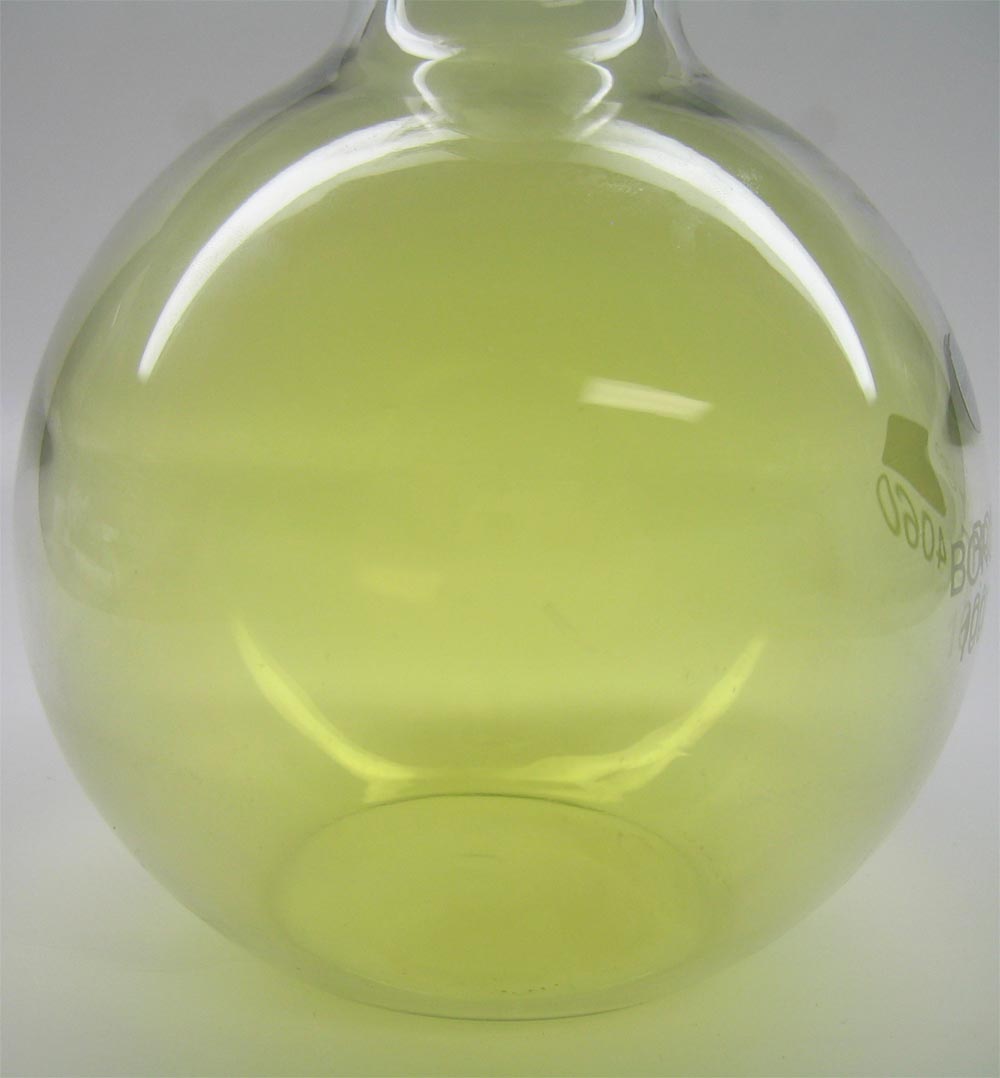This image features a close-up of a spherical glass flask, evocative of a chemistry set or a decorative bottle, containing a yellow, thin liquid. The flask has a neck that extends upwards, though the primary focus is on its round base. Light reflects off the shiny glass surface, accentuating the yellow hue inside, which could be a gas, liquid, or merely colored glass. Stamped letters and numbers, including the reversed reflection of "4060," are visible on the side. The flask also bears a small black logo above the numbering and a silver circle with no inscription on its side. The background is a plain white surface, giving an unobstructed view of the detailed features of the glass orb, which casts a distinctive shine.